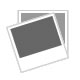The image features a peculiar electronic gadget, which distinctly resembles a handheld scanner or thermometer without a display screen. The device has a silver handle and is equipped with three buttons: two white square buttons and one pink rectangular button. Above the buttons, there's a piece of gray plastic with an opening that reveals a textured background showcasing one reddish stripe and one yellow stripe, adding a touch of color to the otherwise monochromatic device. The top of the device is capped with a black, triangular, plastic protrusion. 

This gadget lies on its side on a weathered wooden surface composed of horizontal planks stretching from the top to the bottom of the image. The wood's condition varies, exhibiting shades of tan with areas showing gray and white wear, indicative of a faded and aged deck.